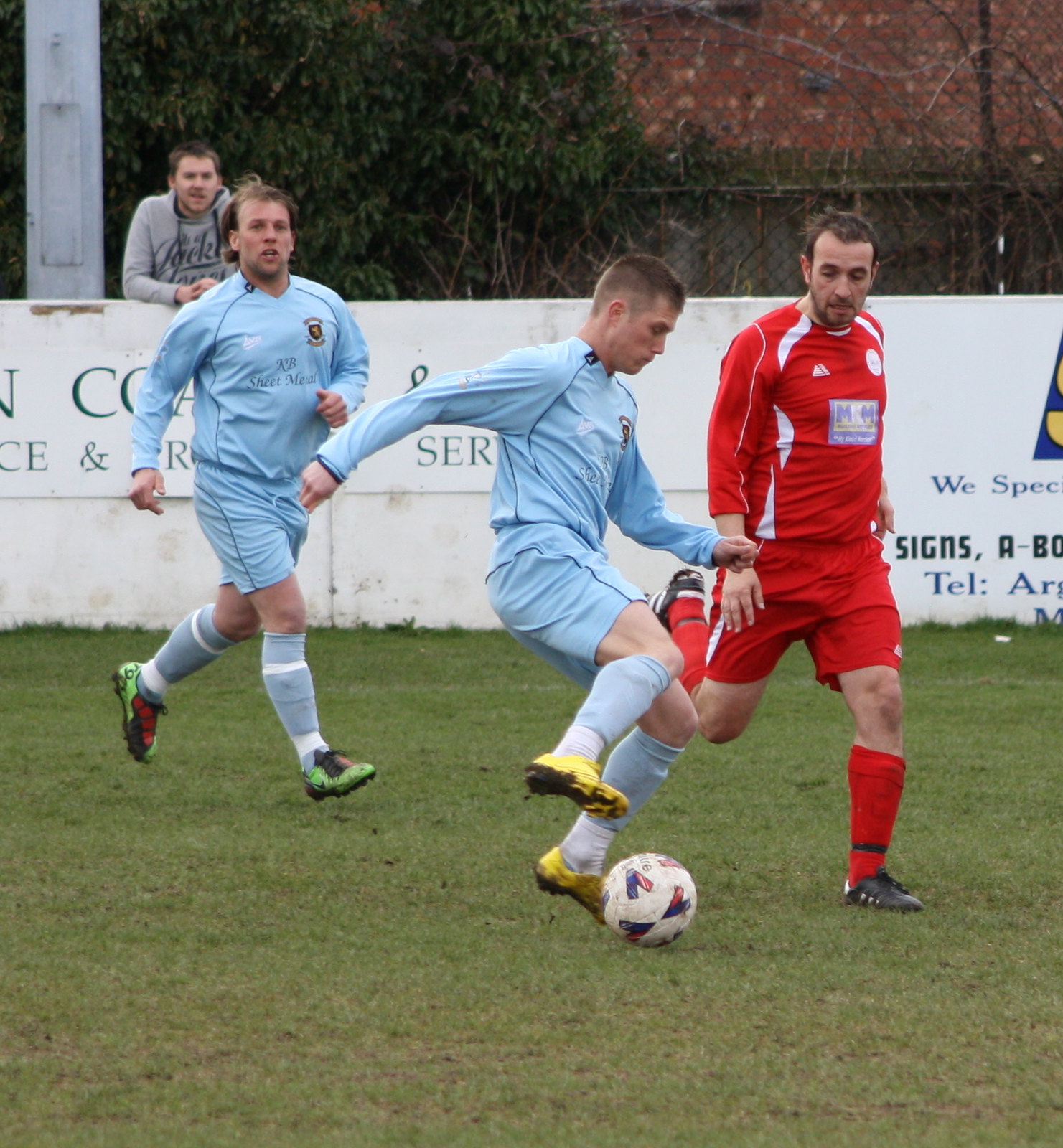This is a daytime, close-up color photograph capturing an intense moment in a soccer game on a grass field. In the foreground, three soccer players dominate the image, positioned from left to right. The two players on the left wear light blue jerseys reminiscent of Manchester City colors, paired with white socks. The player farthest to the left sports green soccer shoes, while the middle player, who is maneuvering a white soccer ball adorned with blue and red shapes, wears yellow cleats. The opposing player on the right is clad in a red uniform with white highlights, complemented by long red socks and black cleats. Behind them, a white wall adorned with advertising signs runs horizontally across the image, partially obscured by the players. Above this wall, a dark green and brick structure is visible. Leaning against the wall, watching the action, is a spectator in a gray hoodie.